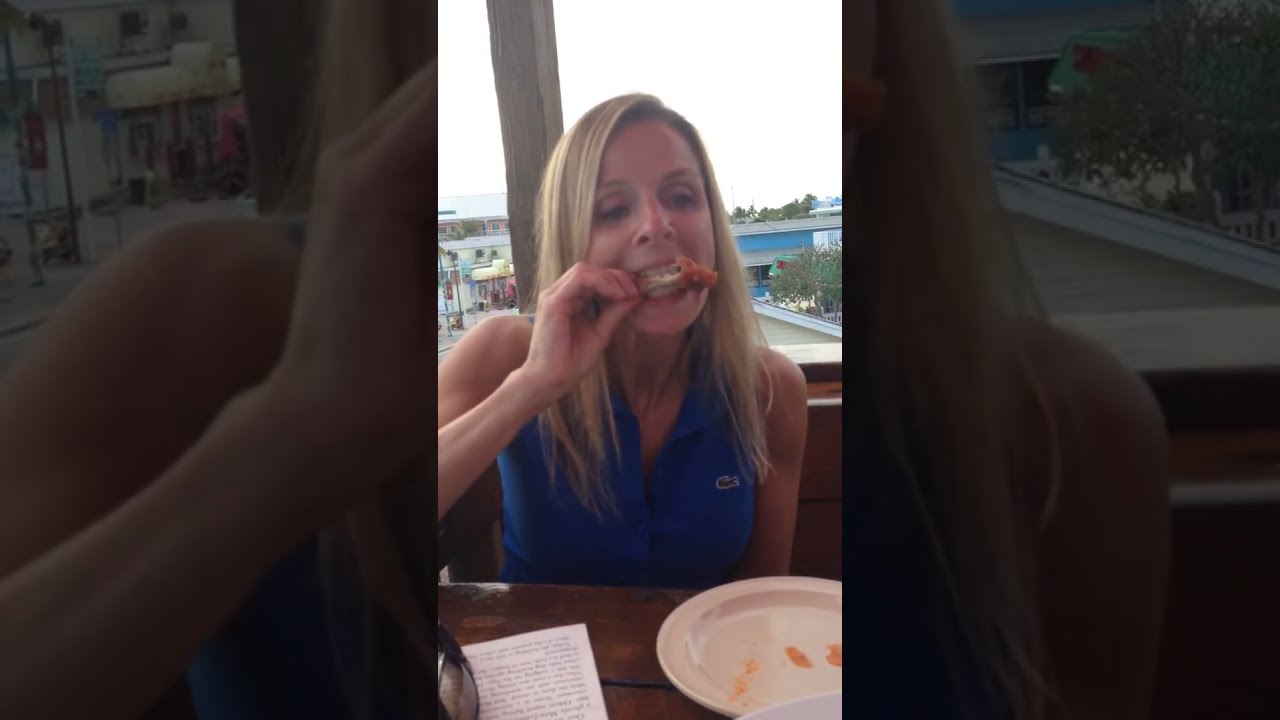The image captures a Caucasian woman, likely in her 40s to 50s, seated in a restaurant booth with a large window behind her, revealing a clear, sunny day outside. The woman has long blonde hair with brunette streaks and a tanned complexion. She wears a blue, sleeveless Lacoste shirt featuring the distinctive crocodile logo on the right side of her chest. Her shirt, resembling a button-down vest with a collar, is partially unbuttoned. 

In her right hand, the woman holds a chicken wing, which she appears to be dipping into some sauce on a white plate placed before her. Her left hand, adorned with a ring on her middle finger, is resting beside the plate. Behind her, you can see buildings, a street, trees, and sections of a blue building, indicating the restaurant is located on an upper floor. The photo, taken in a vertical orientation, focuses solely on the woman as she looks down at her food amidst a warmly-lit, ambient setting.